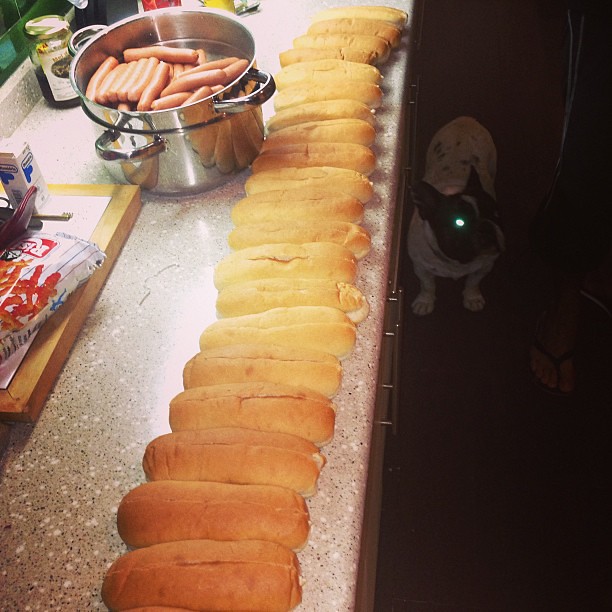This photograph captures a detailed scene of a kitchen countertop prepared for a hot dog feast. Prominently featured is a silver cauldron brimming with flesh-colored, peachy hot dogs. The cauldron, positioned on the left side of the countertop, is adjacent to a row of hot dog buns. These light brown buns stretch from the bottom to the top of the tan marble counter, which is speckled with white and black. To the left of the cauldron sits a wooden cutting board displaying an orange-fronted bag of chips, snack, or possibly french fries, along with a small, partially visible white box adorned with a blue picture. The cutting board has a tile top with a wood rim. In the lower right corner lurks a white and black dog, likely a boxer or bulldog, its left eye glowing from the camera flash. The dog’s face is marked by a white line down the center, interrupted by black splotches, and it sits amidst the shadows cast by the brightly lit countertop. The setting suggests a lively and bustling kitchen preparing for a large meal.